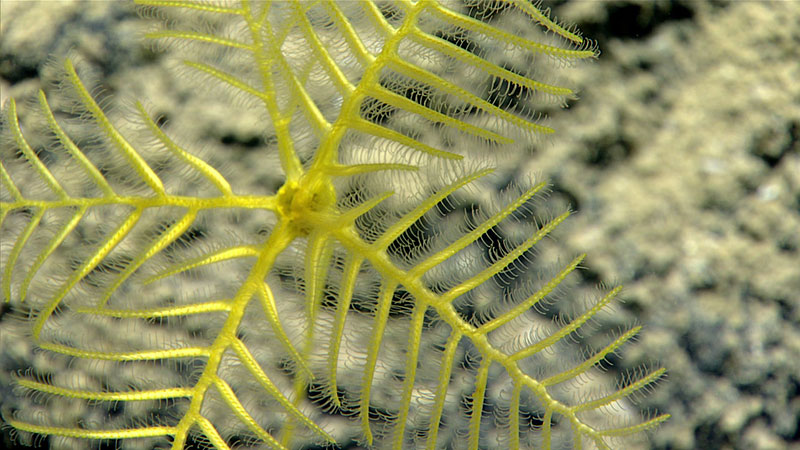This is a highly detailed, macro photograph capturing what appears to be an underwater scene with a yellow, potentially biological specimen at the forefront. The subject of the photo, positioned slightly to the left of the frame, exhibits a fascinating structure reminiscent of a delicate leaf skeleton or possibly the frilled extensions of a sea creature, such as a sea urchin. The central part comprises four leaf-like formations, covered with fine, hair-like tendrils, giving it a somewhat ethereal appearance. These tendrils, or filaments, could suggest a flytrap plant or an underwater organism using them for feeding or movement. The background is a blurred mix of dark greens, blacks, and grays, likely indicating a rocky or coral environment, thereby adding to the mysterious ambiance of the scene. The color palette is dominated by the neon or banana yellow of the central figure, contrasting sharply with the darker, muted tones of the blurred background.